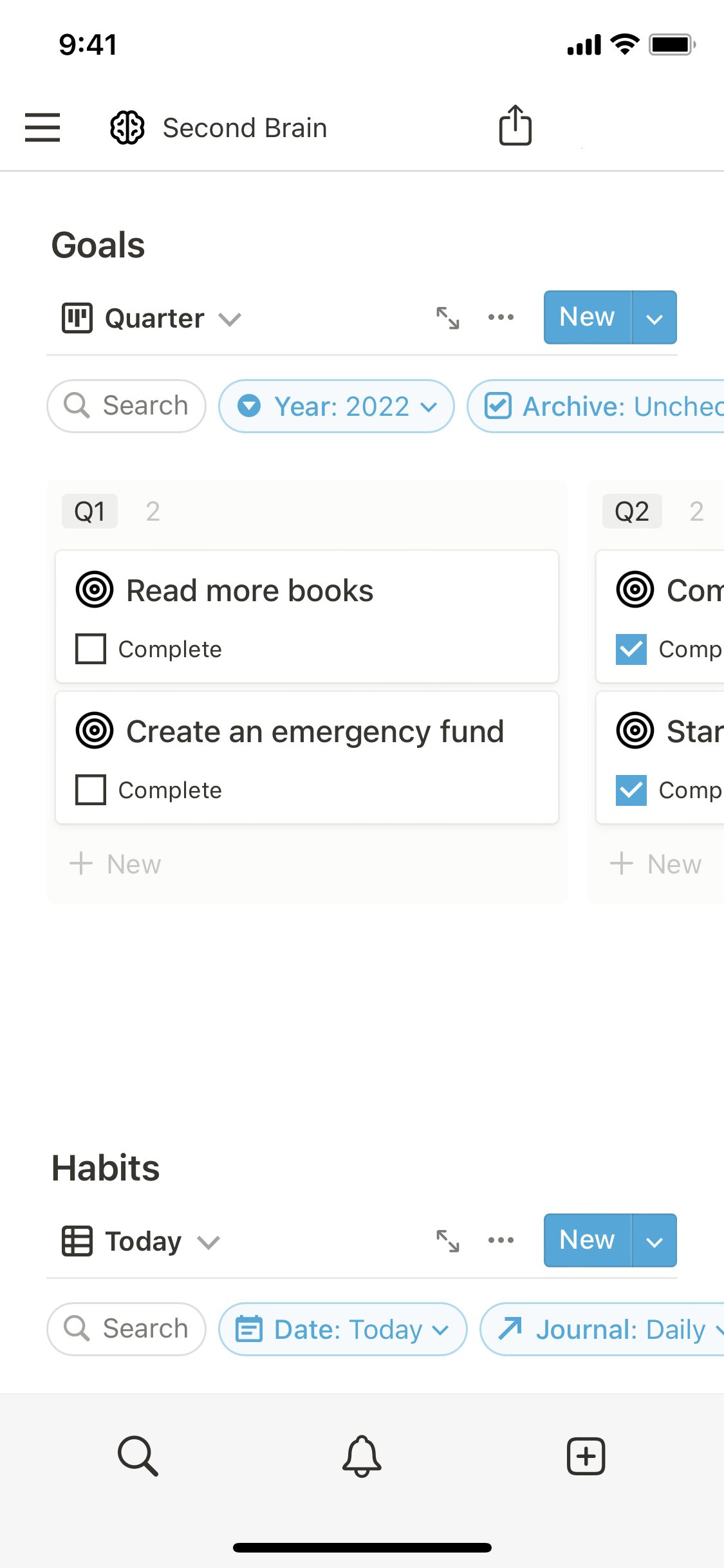This image is a detailed screenshot of a cell phone displaying an organizational app interface. In the upper left corner, the time is shown as "9:41." In the upper right corner, icons indicate strong cellular signal strength, a wireless connection, and a nearly full battery.

At the top section of the app, the title "Second Brain" is prominently displayed. Underneath, the heading "Goals" is featured, followed by the words "Quarter" and "New," suggesting the option to set new quarterly goals.

A dropdown box labeled "Search Year 2022" is present, with a check mark next to "Archive," likely indicating the ability to filter or sort past goals. Below this, "Q1" appears highlighted, signifying the first quarter. 

The section lists individual goals starting with a filled circle labeled "Read more books," paired with an unchecked box and the word "Complete" beside it. This structure repeats for another goal, "Create an emergency fund."

Further down, a "Plus" sign next to the word "New" indicates the option to add more goals. Below this, the "Habits" section appears, with "Today" emphasized and a "New" option to the right.

A search bar, depicted as a magnifying glass with the word "Search," is enclosed in a box. Adjacent to it, dropdown menus display "Date Today" and "Journal Daily," providing quick access to specific dates and journal entries.

The bottom of the app's interface features a light gray background with navigation icons: a magnifying glass in the lower-left corner, a bell icon centrally located, and a square containing a plus sign in the lower-right corner.